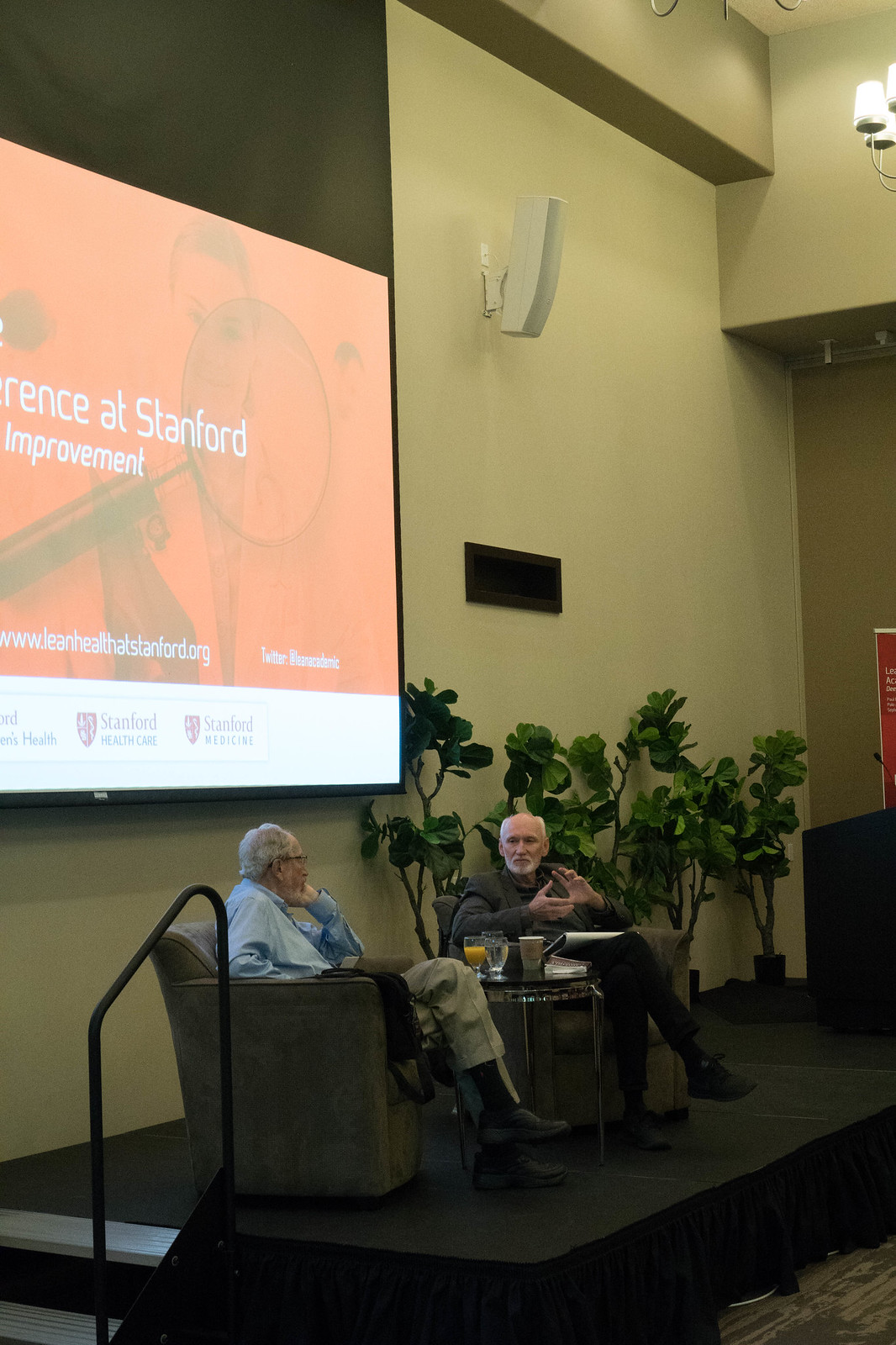The image depicts a conference stage at Stanford, featuring two elderly male speakers engaged in discussion. The stage, which is black with a black skirting, is small and accessible via a set of stairs in the bottom left corner. On the stage, there are four flowerpots and stage lights. The background is beige, contrasting with the gray sofas the speakers are seated on.

The speaker on the left wears a light blue shirt, beige pants, black socks, and black shoes, and has short gray hair. He is turned slightly to his right, facing the other speaker. The speaker on the right, who sports a gray blazer, black pants, black socks, and black shoes, appears to have a white beard and also has short gray hair.

A table with cups and glasses sits between them. Behind them, a large screen displays "Conference at Stanford Improvement" along with the Stanford Healthcare and Stanford Medicare logos. The screen has a red and white color scheme, with a noticeable border at the bottom. The setting suggests the men are in their seventies and possibly conversing with each other and the audience.